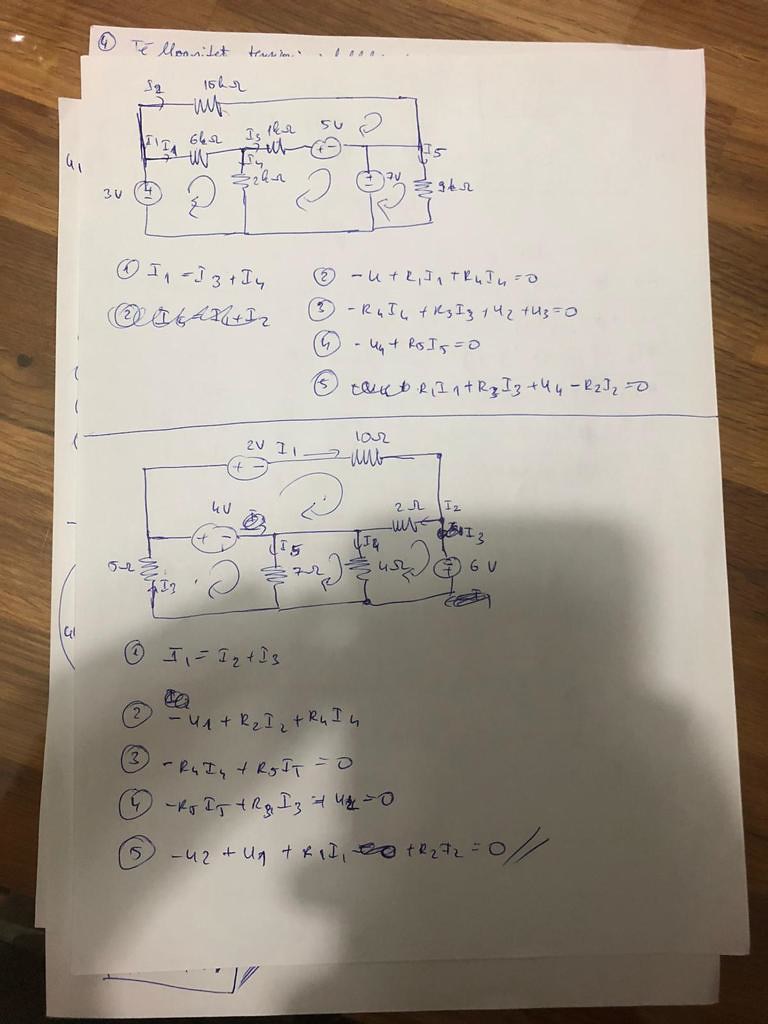A detailed caption for the described image might look something like this:

"A wooden table is strewn with several sheets of white paper, appearing to be someone's math homework. The papers are filled with various mathematical problems, all written in blue ink. Each sheet features multiple boxes, some containing rectangles and squares with meticulously noted measurements along the sides. These annotated shapes suggest that the student is solving geometry problems, focusing on area and perimeter calculations. Below these shapes, there are two sets of squares separated by a line, each with numbers (1, 2, 3, 4, 5), where the initial '2' is crossed out and rewritten. Each number is circled, accompanied by corresponding formulas. The student’s handwriting is somewhat messy, making the formulas difficult to decipher, yet presumably clear to them. In the lower part of the image, more rectangles adorned with extensive writing and formulaic notations can be seen, indicating detailed problem-solving steps. The shadow of a person holding a phone to take this picture stretches across the paper, adding a human element to this study scene."